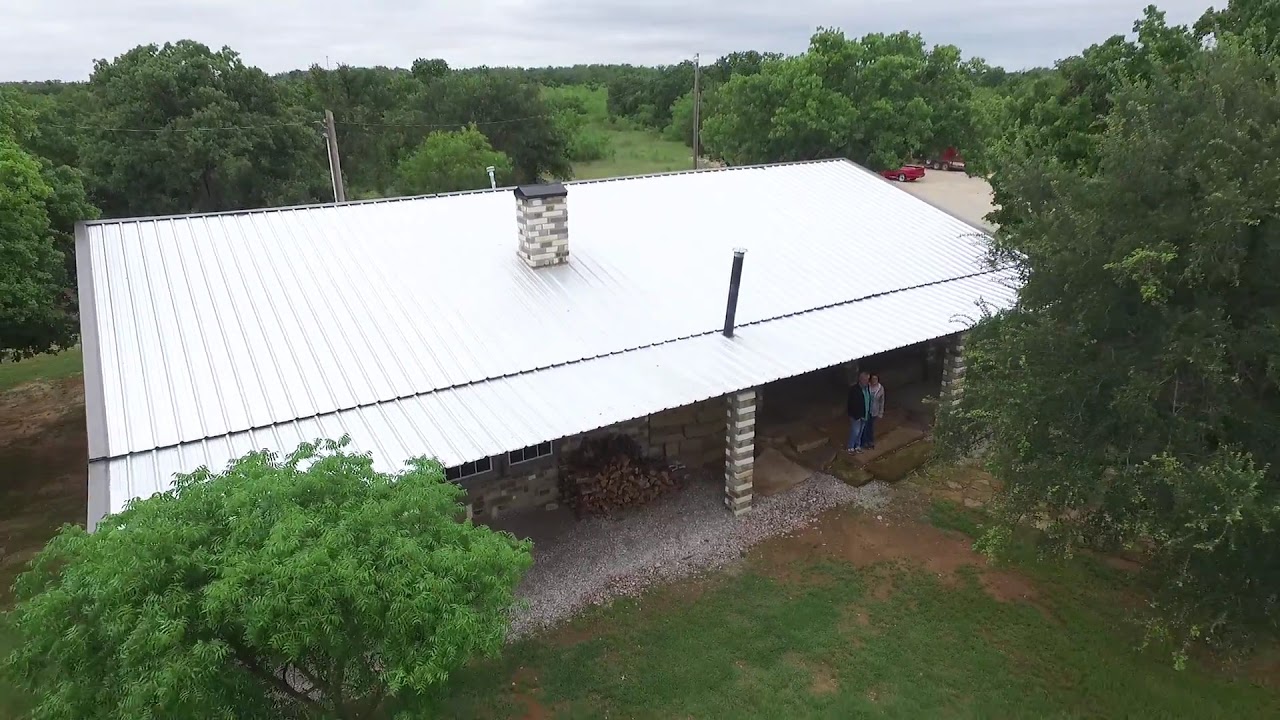The image depicts a countryside scene looking down from a height of approximately 25 feet onto a building with a white metal roof and a white and gray brick chimney positioned at its center. There are vertical support columns at the base, suggesting a roof overhang. The building, which could be a cabin for camping, features a stone facade with a few visible windows on the left side and possibly a woodpile stacked against the stone wall. Two people, a male and female, stand under the awning near a wood entryway; one wears a jacket and the other a light-colored shirt and light blue jeans. The surrounding area is rural, with green grass and various trees encircling the structure. In the background, there's a parking area with at least one red vehicle visible. A telephone pole and wire stretch into the partly cloudy, gray sky.